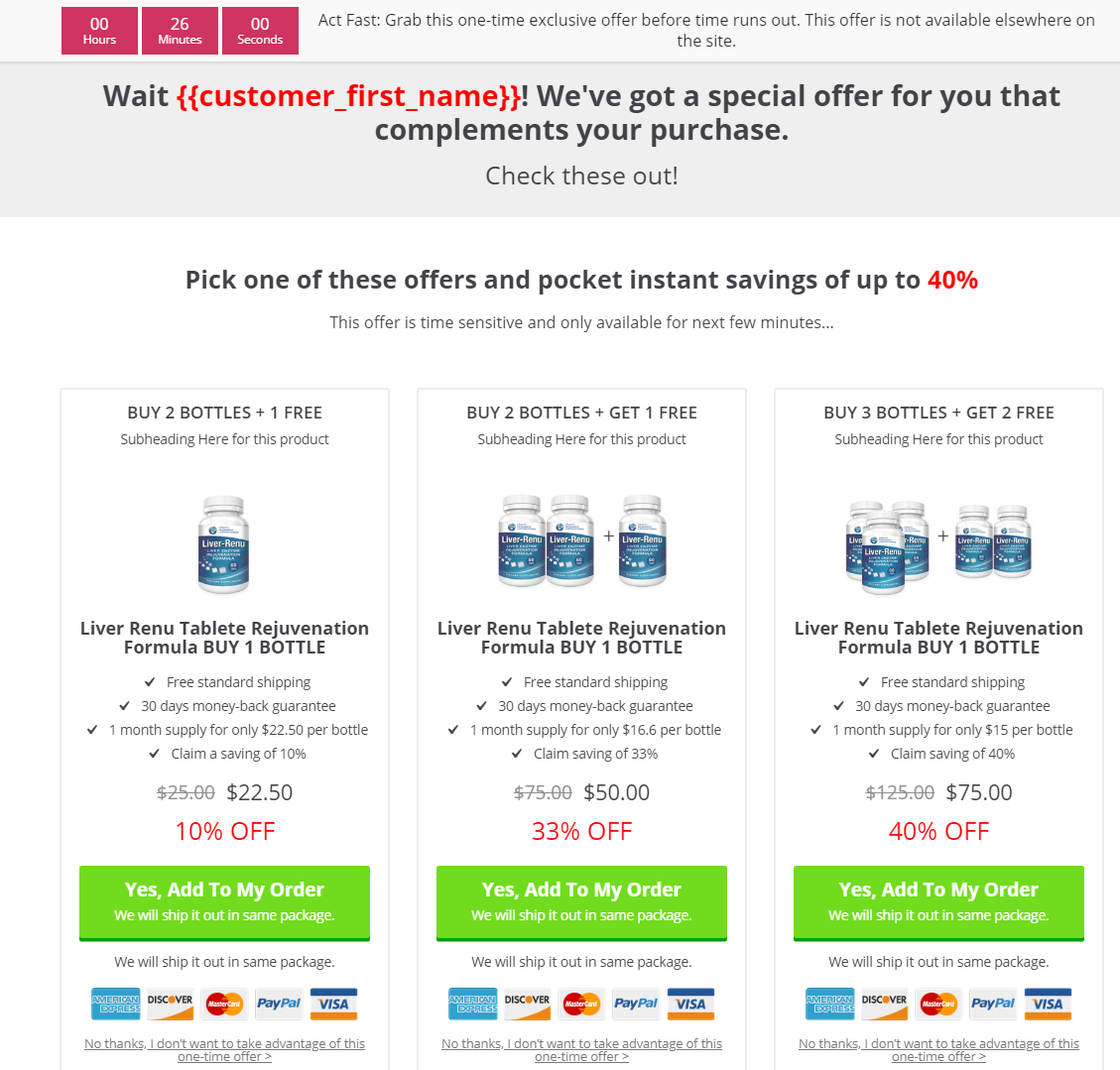The screenshot captures a promotional page from a vitamin website, offering a limited-time deal on their products. At the top, against a white background, there are three adjacent red squares displaying time in hours, minutes, and seconds in white font. To the right of these squares is text urging customers to "Act fast, grab one of these time-exclusive offers before time runs out."

Directly below, a rectangular gray area addresses the customer by their first name, stating, "Wait, [Customer's First Name]. We've got a special offer for you that complements your purchase. Check these out."

Further down, the background remains white and the page promotes three products with a headline: "Pick one of these offers and pocket instant savings up to 40%," with "40%" highlighted in red. Below this are three vertical rectangles, each detailing a different offer:

1. **Left Rectangle:**
   - Product: Liver Renew Tablets
   - Offer: Buy two bottles, get one free
   - Discount: 10% off (in red at the bottom)
   - Purchase Option: Green rectangular button with white text, "Yes, add to my order. We will ship it out in the same package."
   - Payment Options: Logos of American Express, Discover, MasterCard, PayPal, and Visa
   - Opt-out: Text stating, "No thanks, I don't want to take advantage of this one-time offer."

2. **Center Rectangle:**
   - Product: Liver Renew Tablet Regeneration Formula
   - Offer: Buy one bottle, get two free
   - Discount: 33% off (in red at the bottom)
   - Purchase Option: Green rectangular button with white text, "Yes, add to my order. We will ship it out in the same package."
   - Payment Options: Logos of American Express, Discover, MasterCard, PayPal, and Visa
   - Opt-out: Text stating, "No thanks, I don't want to take advantage of this one-time offer."

3. **Right Rectangle:**
   - Product: Liver Renew Tablets Formula
   - Offer: Buy three bottles, get two free
   - Discount: 40% off (in red at the bottom)
   - Purchase Option: Green rectangular button with white text, "Yes, add to my order. We will ship it out in the same package."
   - Payment Options: Logos of American Express, Discover, MasterCard, PayPal, and Visa
   - Opt-out: Text stating, "No thanks, I don't want to take advantage of this one-time offer."

This detailed promotional structure is designed to entice the customer with various bulk purchase discounts, highlighted savings, and simple call-to-action buttons, all supported by various secure payment options.